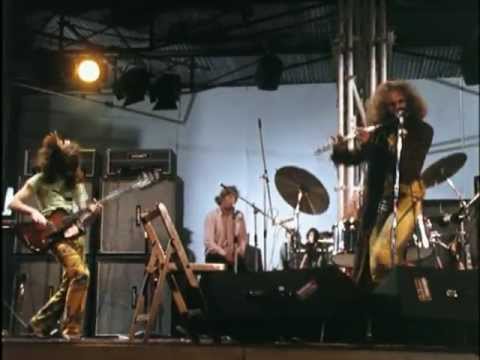This photograph captures a grainy and slightly blurred snapshot of a rock band performing live on stage, likely from the 1970s judging by the styling and quality. To the right, a frontman, dressed in a dark jacket, is playing a flute with a microphone stand in front of him, reminiscent of Ian Anderson from Jethro Tull. On the left, another musician is energetically playing a red and black electric guitar, his long hair obscuring his face, and he is clad in a t-shirt. Behind them, a drum set and cymbals are visible, although the drummer himself is not in the frame. A person in a pink jacket is seated on a fold-out chair next to the stage, adding to the casual vibe of the scene. Large stacks of amplifiers dominate the background, enhancing the rock concert atmosphere. A singular, intensely bright stage light in the upper left corner illuminates the otherwise dimly lit and muted environment, contributing to the raw and unpolished feel of the photograph.